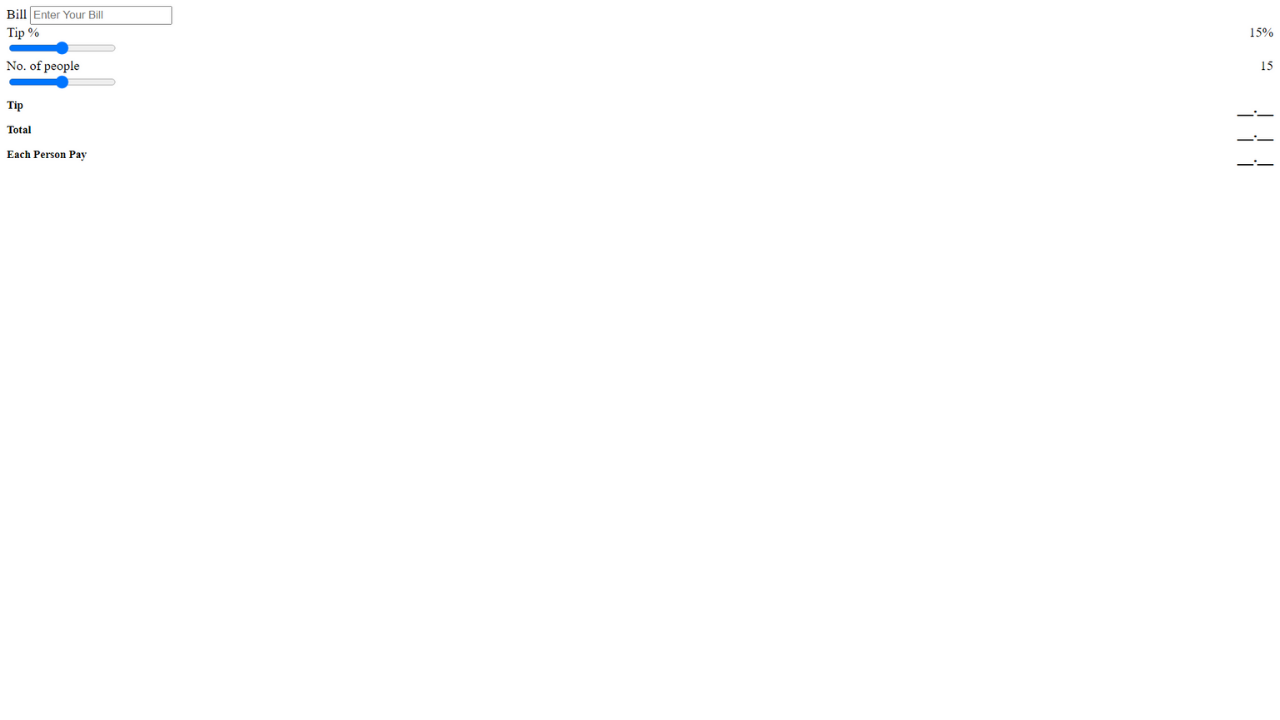The image depicts a white background with text and input fields associated with a bill and tip calculator. At the top, it has the word "Bill." Below this, there is a box labeled "Enter your ID" and another labeled "Tip Percent" accompanied by a blue slider. Underneath, there is a section labeled "Number of People" with another blue slider. Subsequently, there are fields marked "Tip," "Total," and "Each Person Pays." The bottom part of the image contains some indistinct elements, including faint, swirling lines and barely visible black numbers. On the right side of the image, percentage options are listed: 15%, 25%, and three smaller, illegible options.